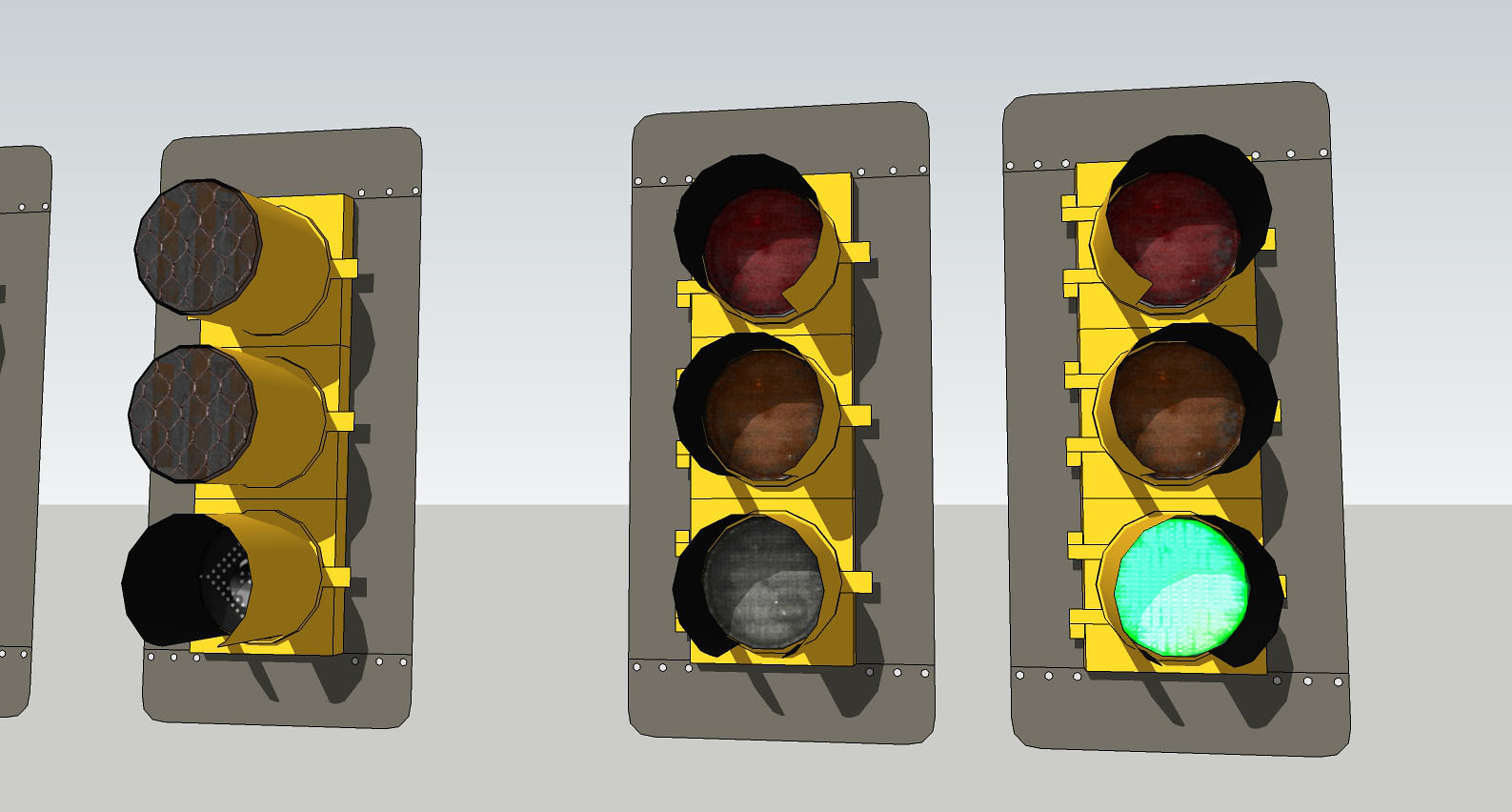This image features a detailed graphic of three vertical traffic lights mounted on a wall. The background is divided horizontally, with the upper half in a light gray and the lower half in a darker gray. Each traffic light is affixed to a dark gray vertical rectangular board and secured on yellow platforms.

The left-most traffic light has yellow paint with its top two lenses covered, leaving the bottom lens uncovered but not illuminated. The middle traffic light similarly has three vertical lenses: red at the top, yellow in the middle, and green at the bottom, although none are lit. The right-most traffic light is also painted yellow with three vertical lenses, but only the bottom lens is lit up in a bright neon green, indicating "go," while the top red and middle yellow lenses are off.

The setup appears to be a design drawing or a generated image rather than an actual photograph. The traffic lights are possibly part of an art project or testing environment, as they are bolted to the wall and not situated on a street. Additionally, the image hints at the presence of a partial fourth traffic light on the left edge, suggesting more lights outside the visible frame. Overall, the scene conveys a controlled, indoor setting possibly aimed at testing or showcasing traffic light designs.